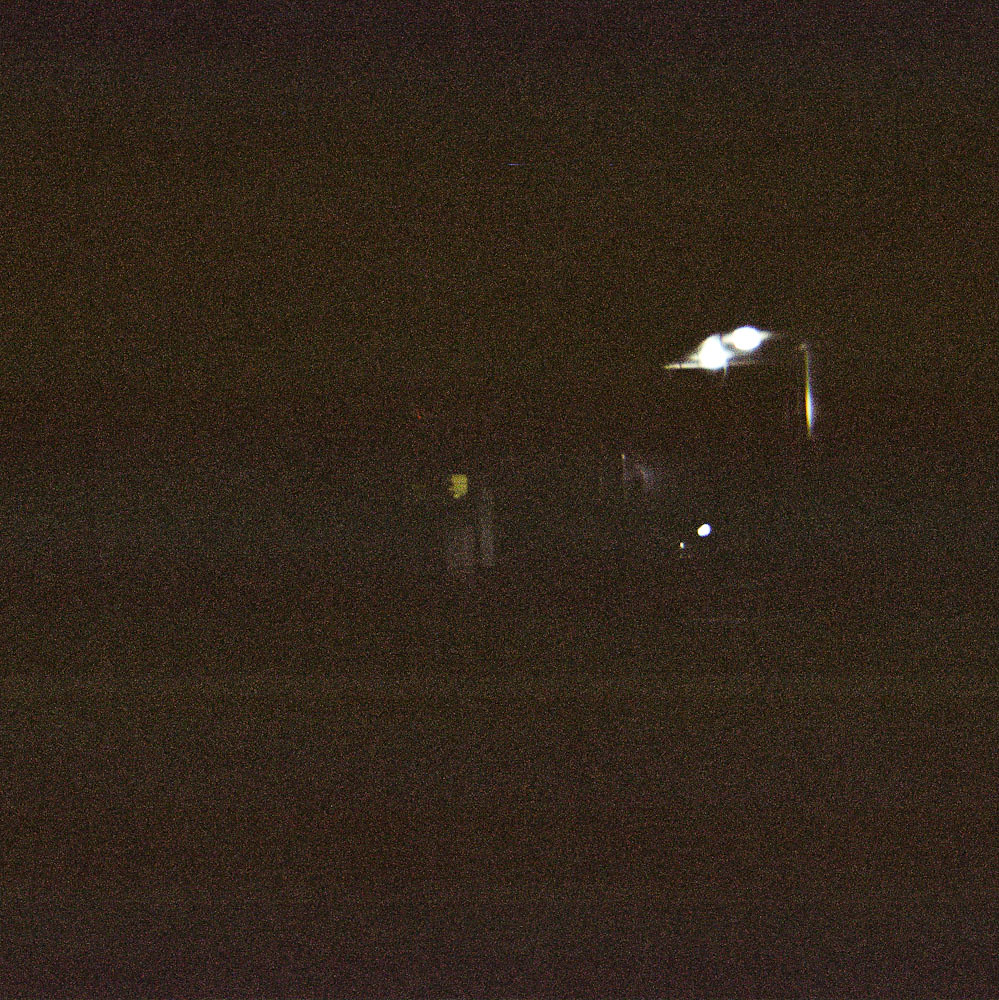This outdoor color photograph, taken at night, captures a scene shrouded in darkness with limited visible details. Left of center, there appears to be a faint outline of a doorway belonging to a one-story building. To the right of center, slightly upwards towards the top right corner, two white street lamps cast their light downward, creating a slight reflection on the vertical pole supporting them. Beneath and to the right of these lamps, a smaller white light is also visible. The lower portion of the image reveals a dim horizontal line, which may represent the curb of a street or a sidewalk, stretching from left to right. The overall graininess and obscurity of the photograph suggest it was taken on a dark, possibly moonless night, offering a mysterious glimpse of what could be a house beside a road. No words or text are present in the image, adding to its enigmatic quality.